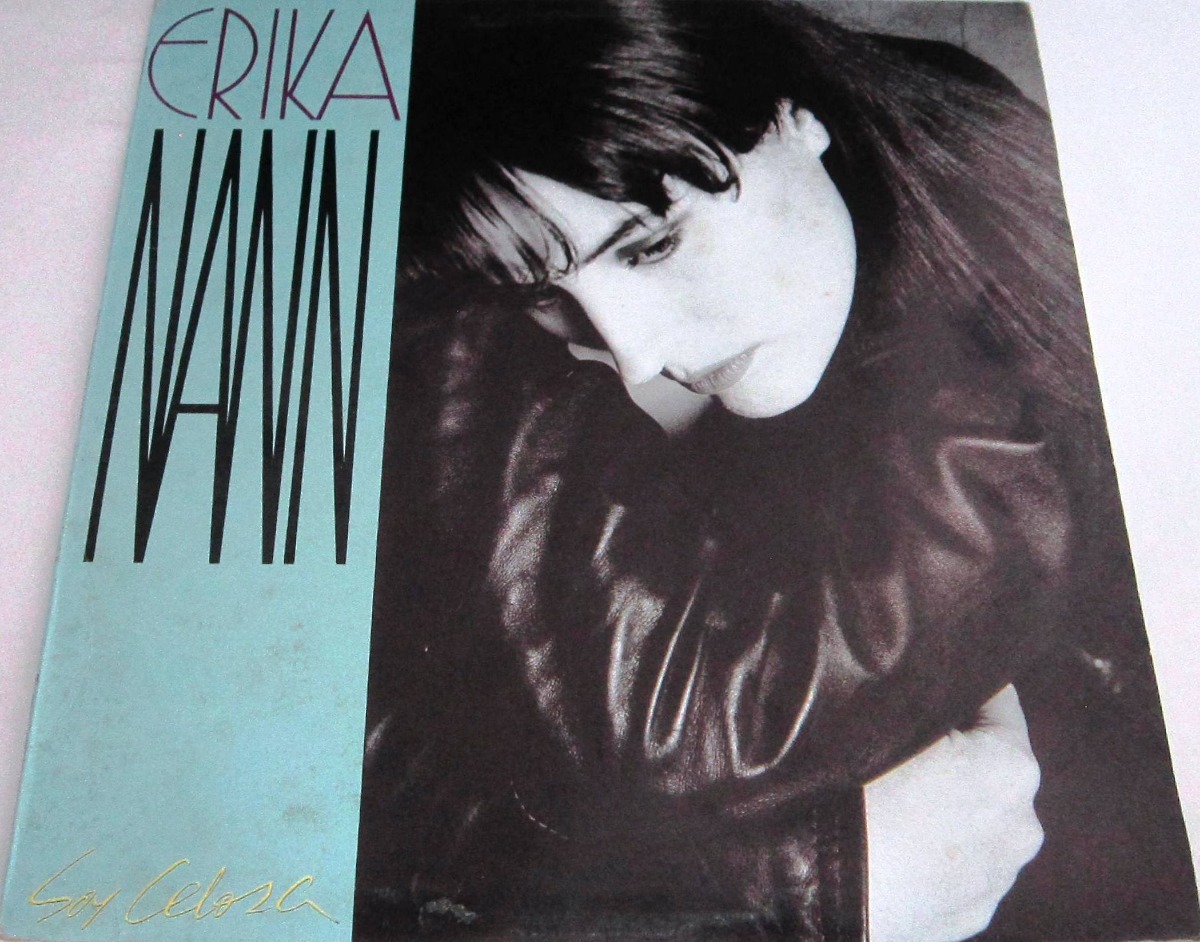The image depicts an album cover with a distinct design and emotional portrayal. On the right side, a black-and-white photograph captures a woman, likely the singer, who appears to be hugging herself, conveying a sense of introspection or sadness. She is hunched forward, with dark hair flowing down her back, prominent bangs brushing her dark eyebrows, and shadowed eyelids accompanying her dark eyes. Her lips bear some color, indicating subtle makeup. She wears a black leather jacket, with one of her hands visible under her arm. The woman, with fair skin, gazes pensively off to the side.

On the left side of the album cover, a vertical sea-green bar runs from top to bottom, set against the grayish surface upon which the cover rests. In thin purple letters at the top, it reads "Erica," followed by "Nan," spelled as N-A-N-N, in bold black oblong letters. At the bottom of the green bar, the title "Soy Celosa" is written in thin yellow letters, adding an additional layer of detail to the overall composition. The image angle suggests a slight slant, enhancing the dynamic presentation of the cover.